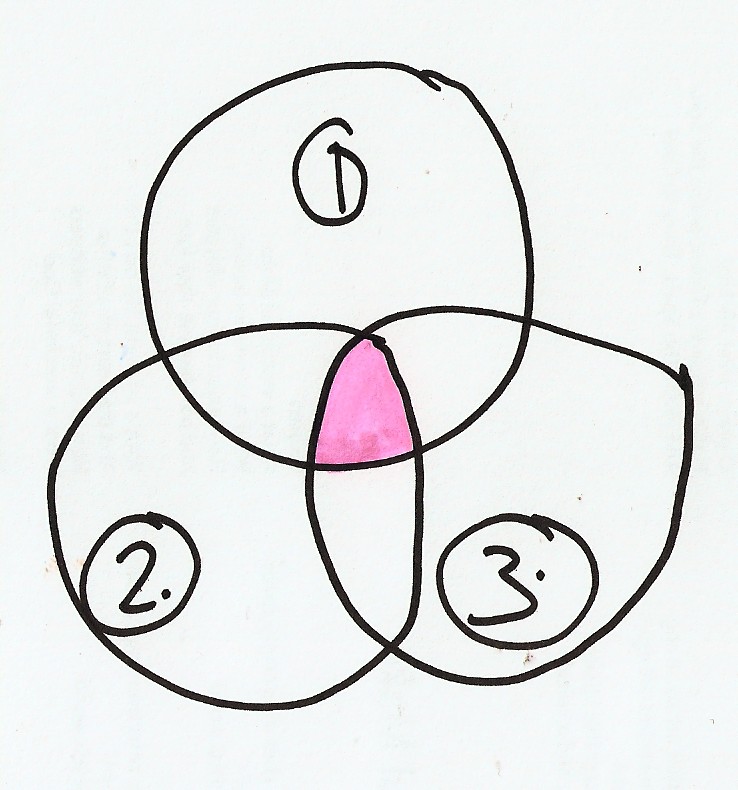The diagram is a meticulously hand-drawn Venn diagram created with black ink on very pale greenish-blue paper. It features three circles, each intricately overlapping the others. The circles are labeled as Circle 1, Circle 2, and Circle 3. Circle 1 intersects with both Circle 2 and Circle 3, forming a central region where all three circles overlap. This area of intersection is highlighted with a pink coloration, drawing attention to the commonality shared among the three sets. This Venn diagram visually represents the relationships and common elements among the data sets delineated by the three circles, a tool frequently employed in mathematics for such analyses.